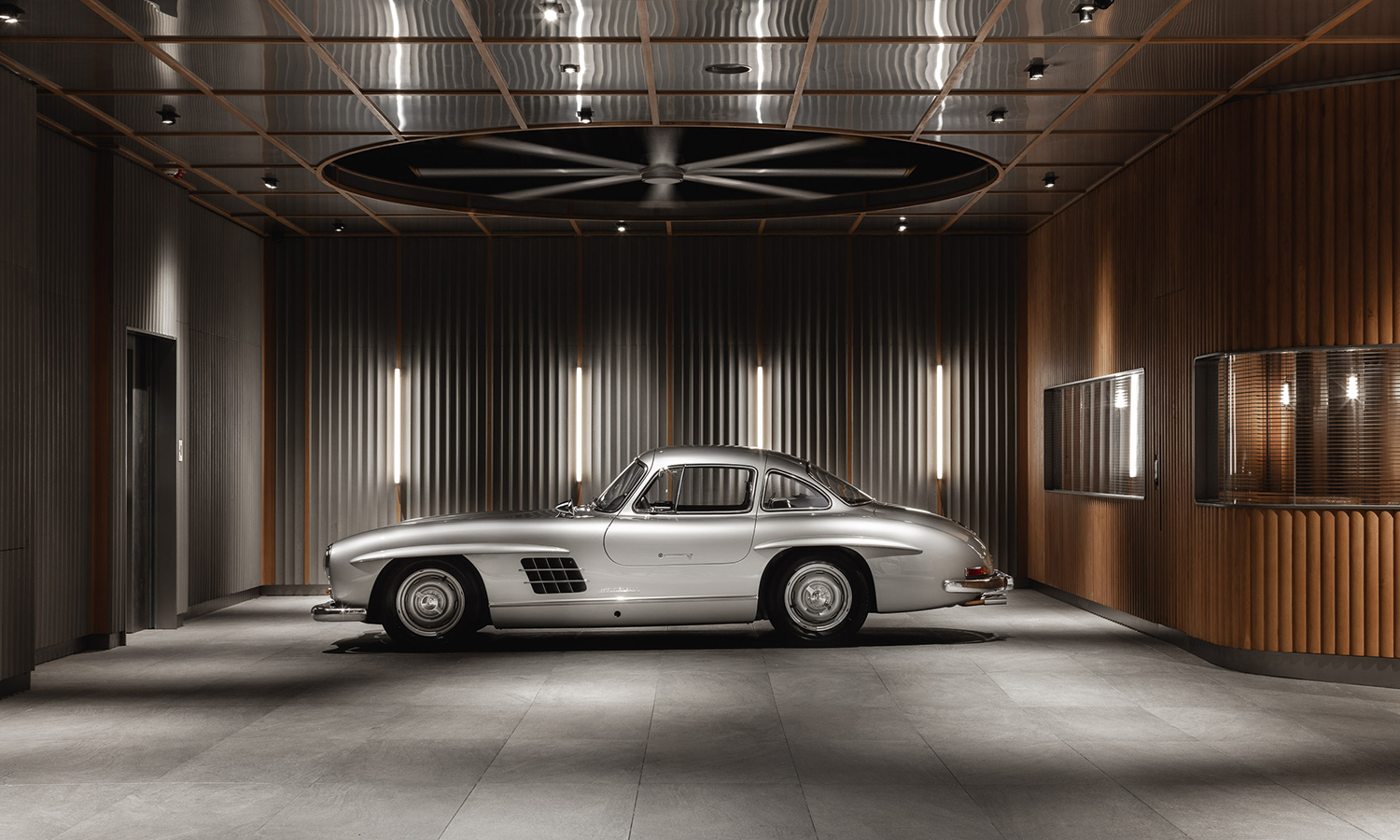The photograph captures a stunning vintage sports car, resembling a 1960s or 1970s model, possibly an Aston Martin, reminiscent of the iconic James Bond vehicles. The car features a sleek silver exterior with elegant curves and a two-passenger setup, boasting silver hubcaps with black tires, and silver bumpers on both the front and rear. This side-view image showcases the car with its front pointed to the left, set inside an opulent showroom space. The interior displays gray tiled floors, gray walls with vertical lights, and a striking ceiling fan with a silver rectangular grid pattern. To the right of the image is a distinctive curved wooden wall with multiple windows, and four vertical light sections in the background, while to the left, a door or elevator entrance is visible. This luxurious setting suggests a high level of security, befitting such a magnificent and well-preserved automobile.